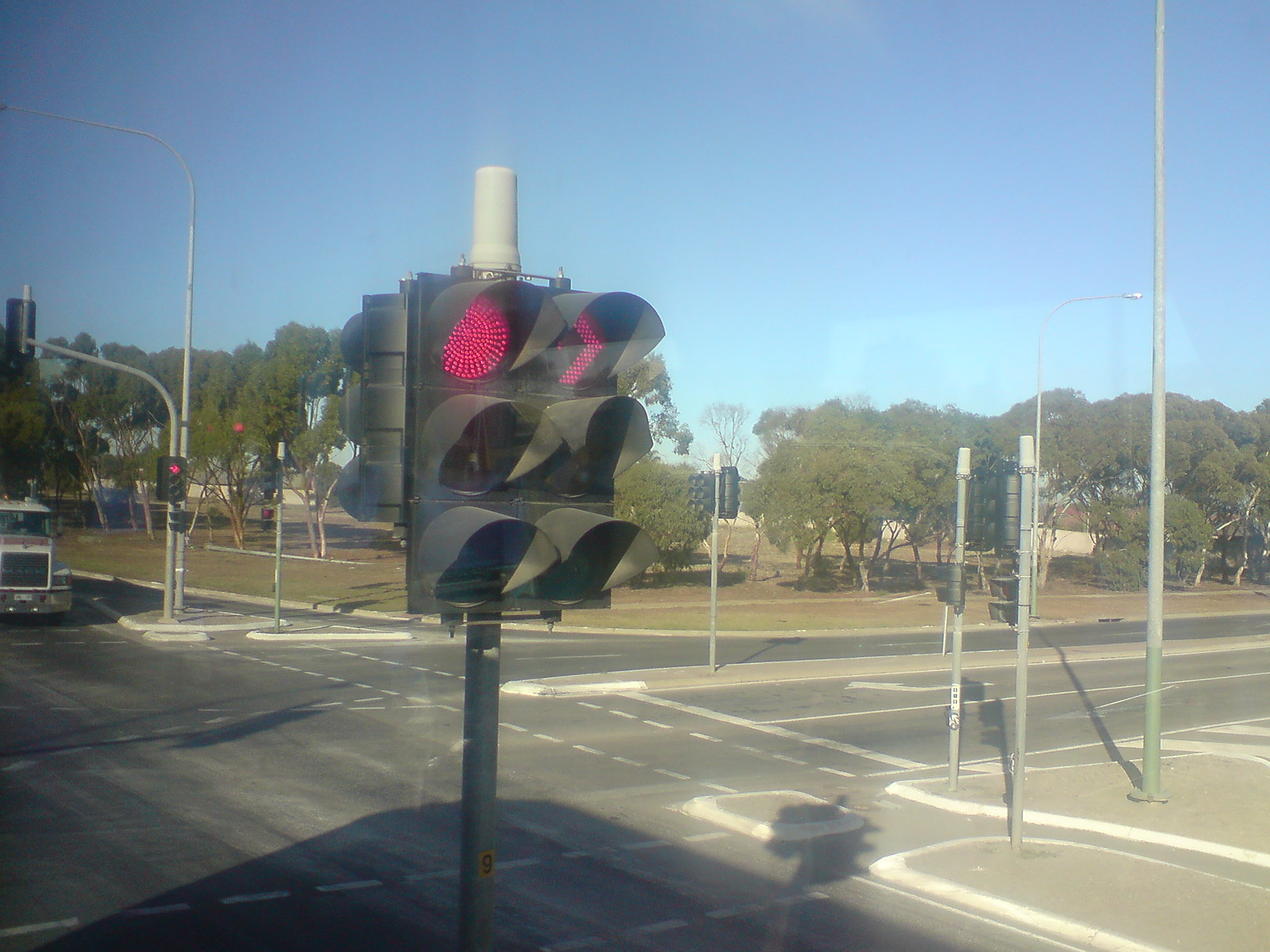The photograph captures a large intersection under clear blue skies, featuring prominently two red traffic lights mounted side by side on a black pole in the foreground. One light displays a red circle, while the adjacent light shows a red arrow. The intersection itself is devoid of cars, except for a white semi-truck visible in the background, stopped at the light. Trees surround the area, suggesting the presence of a nearby park. The image appears to have been taken through a window, resulting in a slightly blurry quality, and reveals long shadows in the scene, hinting at taller buildings behind the perspective of the camera. The intersection is well-marked with crosswalks and turn lanes, contributing to the sense of it being a vast and organized traffic junction.